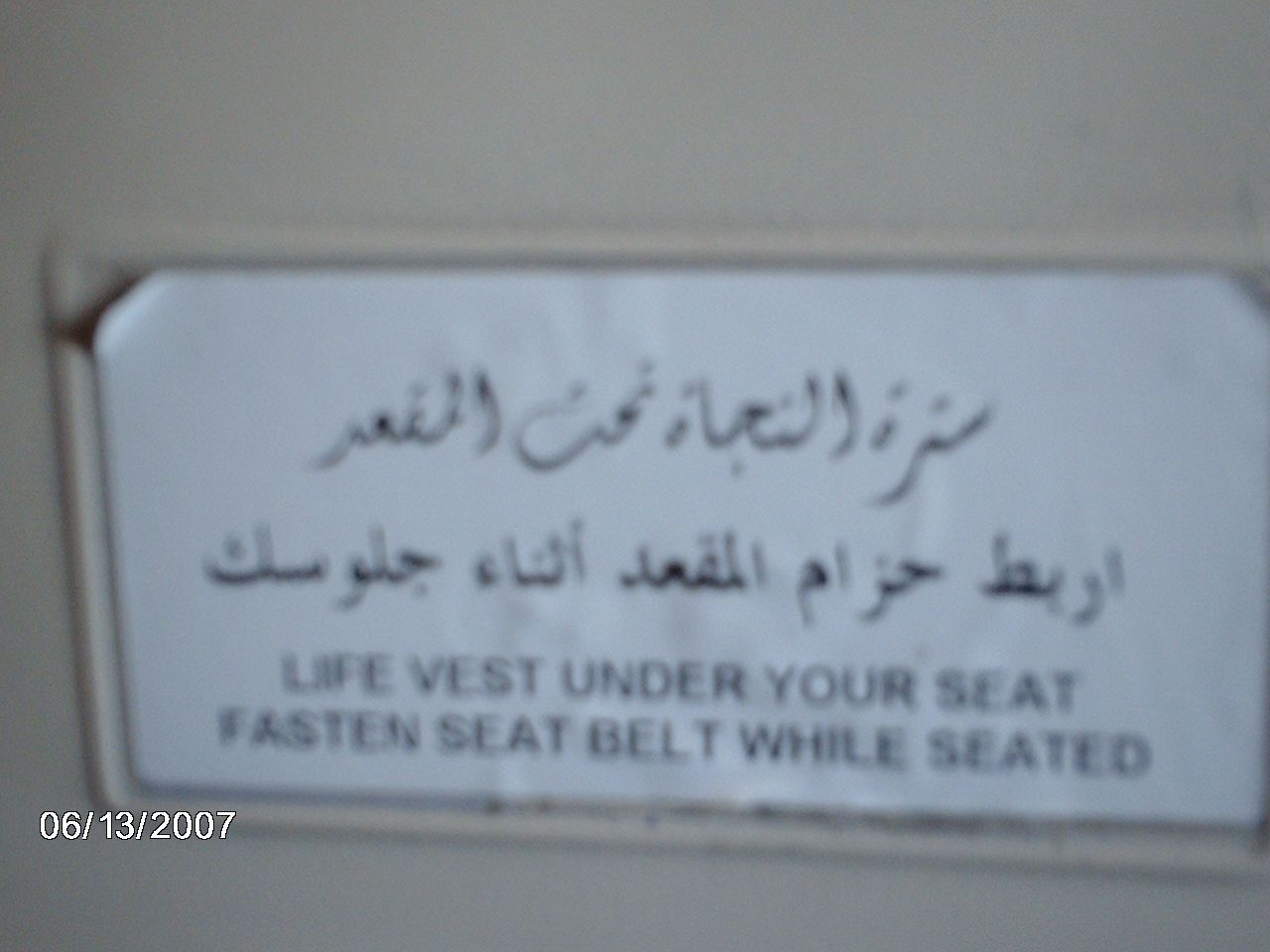This image features a slightly out-of-focus sign mounted against a tan background, likely on an airplane or another moving vehicle. The sign has a rectangular shape with a raised border, suggesting it’s a designated informational sticker. The top half of the sign contains text in Arabic, followed by a possible continuation of Arabic, or perhaps Farsi, script. Below this, in English, it reads: "Life vest under your seat," and beneath that, "Fasten seat belt while seated." The sign itself is white with black text, which contrasts against the tan background. In the bottom left corner of the image, there is a watermark displaying the date 06/13/2007.